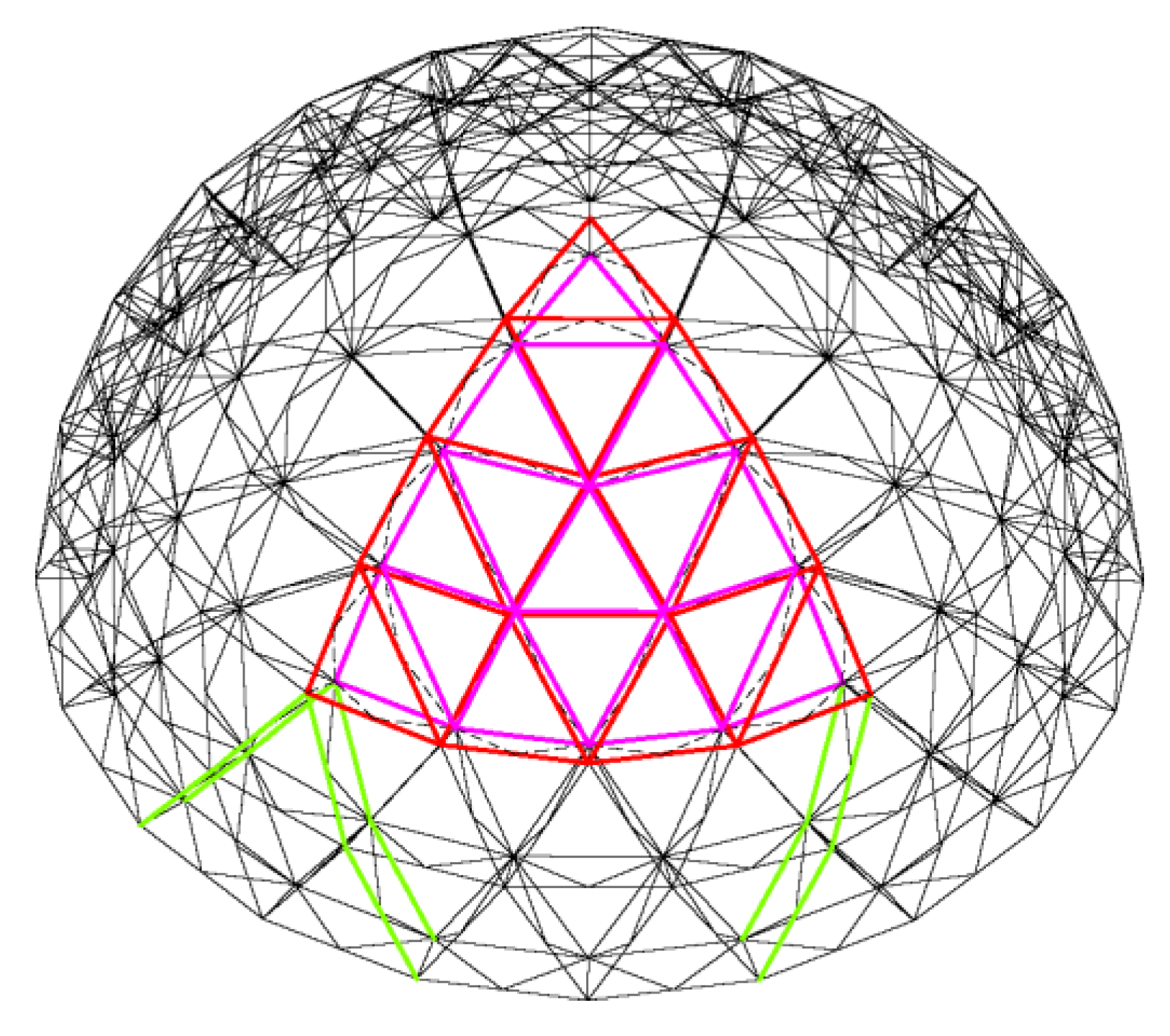This image features a geometric pattern that appears to merge spherical and polygonal elements. The overall shape is somewhat spherical but closely resembles an octagon, characterized by a web of interlocking black lines forming a complex, mesh-like structure reminiscent of computer animations. The black lines are thicker at the top, creating a spider-web effect, while near the bottom, these lines transform into a series of interconnected diamond shapes.

Dominating the center of the image is a large, almost triangular shape with a slight rounding at the bottom, rendered in shades of purple-pink. Within this primary triangle lies a smaller, intersecting red triangle, creating an intricate pattern of multiple connected triangles. This central structure gives the impression of an overlapping or dual-layered image rather than separate triangles positioned in different spatial planes.

Accenting this central design are green lines that run vertically along both sides of the shape, tracing the contour of the triangles and reinforcing the interconnected pattern. Additionally, there are subtle blue dotted lines weaving through the top and bottom sections, adding to the intricate and layered appearance of the composition. The overall effect is a harmonious blend of spherical forms and triangular configurations, unified by their shared geometric intricacies.